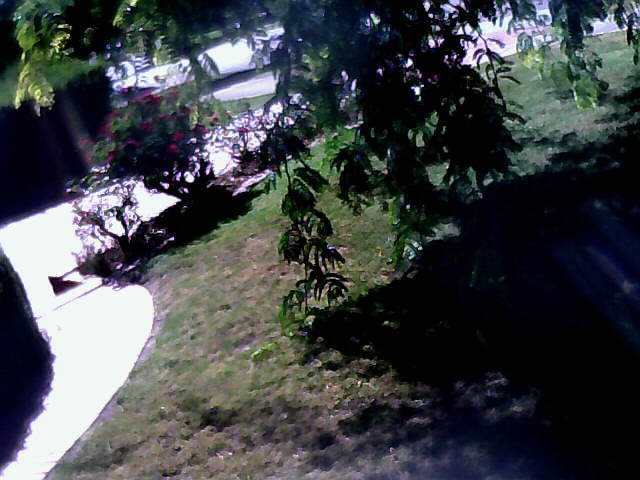This photo, although blurry and poorly lit, captures a scene with various distinct elements. In the foreground, a glowing sidewalk shimmers under a filter-like light, reflecting an eerie, almost dreamlike quality. Adjacent to the sidewalk, there's a yard dominated by a large tree, whose limbs droop almost to the ground, casting deep shadows beneath it. Beside the sidewalk stands a smaller tree, resembling a rose bush adorned with vibrant red blooms. In the background, a structure or object with a grassy or green roof, or perhaps a tree with a remarkably flat top, is partially visible. Further back, a stretch of asphalt driveway leads to a street. Under the large tree, there's a blue tent positioned within a bare patch where the grass is missing. The overall mood is one of a surreal, shadowy day.